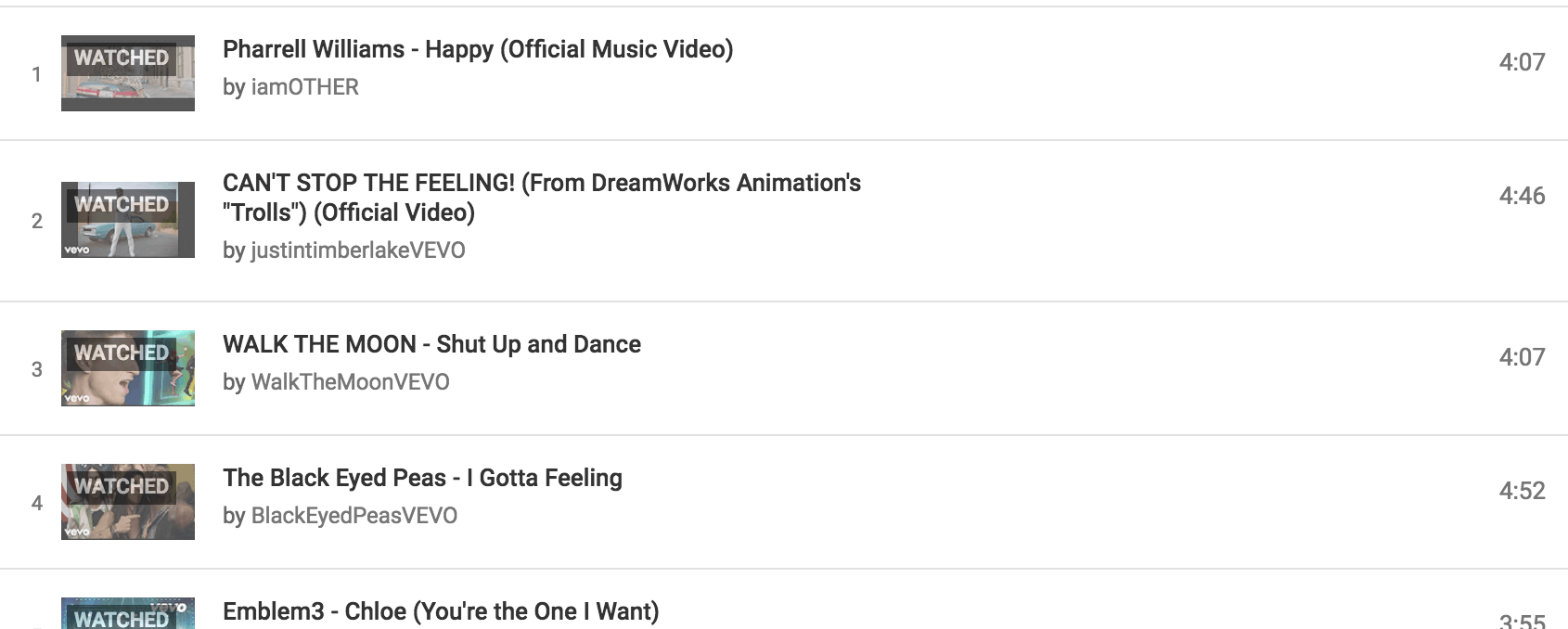This image displays a YouTube playlist featuring a series of music videos, each marked with a "watched" overlay indicating they have already been viewed. The playlist includes the following entries, enumerated sequentially from one to four:

1. **Pharrell Williams - "Happy" (Official Music Video)**: This video, lasting 4 minutes and 7 seconds, is uploaded by the channel "I Am Other."
 
2. **Justin Timberlake - "Can't Stop the Feeling"**: Featured in DreamWorks Animation's "Trolls" official video, it has a duration of 4 minutes and 46 seconds and is hosted on the Justin Timberlake Vevo channel.
 
3. **Walk the Moon - "Shut Up and Dance"**: Running for 4 minutes and 7 seconds, this video is available on the Walk the Moon Vevo channel.
 
4. **The Black Eyed Peas - "I Gotta Feeling"**: This music video, from the Black Eyed Peas Vevo channel, lasts for 4 minutes and 52 seconds.

The playlist also includes a partially visible fifth video:
- **Emblem3 - "Chloe (You're the One I Want)"**: This video, which has been watched, is 3 minutes and 55 seconds long, though the full details are obscured.

The textual elements on the playlist are presented in black font against a white background, with thin black lines delineating each video entry to clearly separate them.